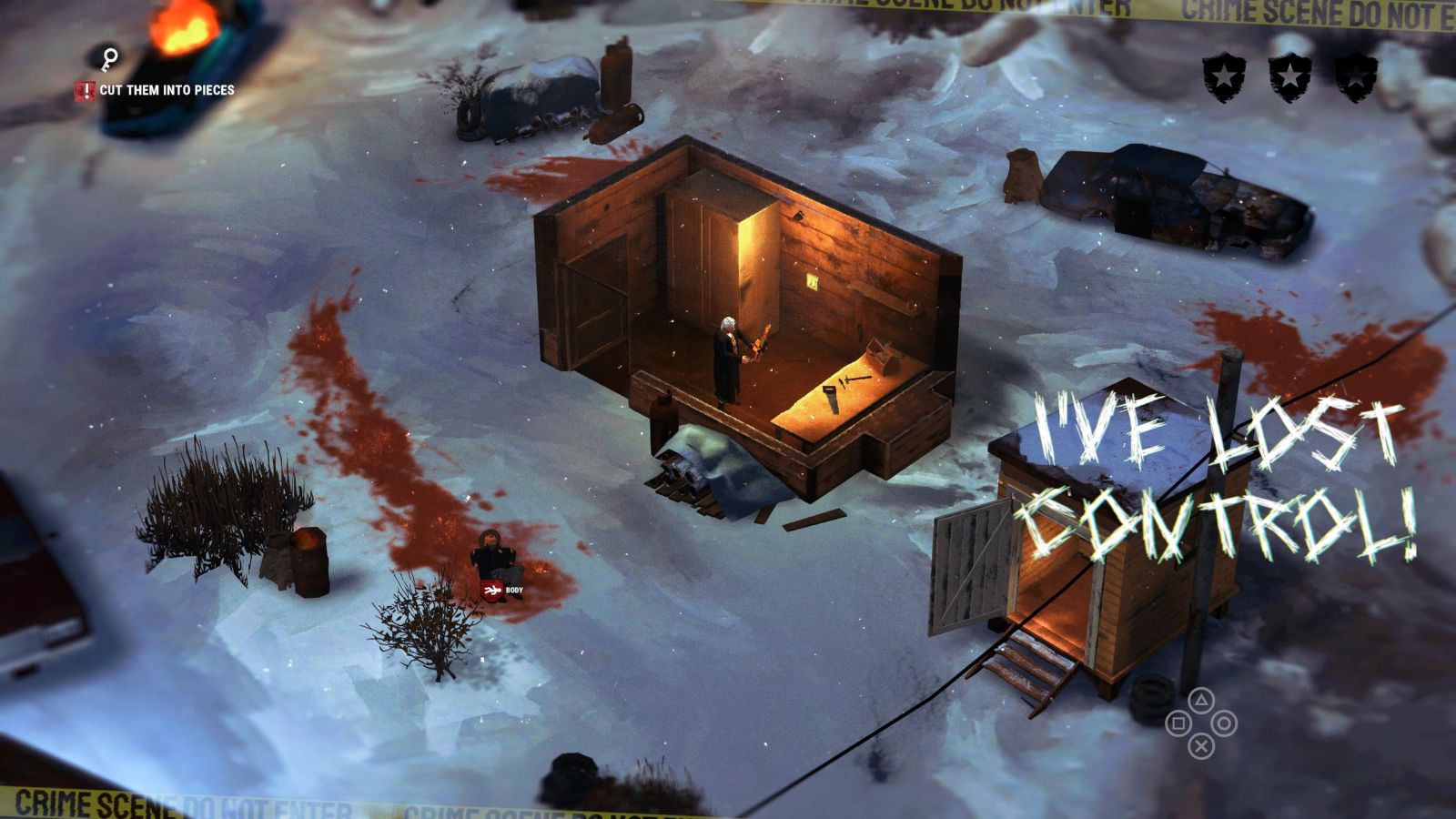The image is a detailed screenshot from what appears to be a video game, depicting a miniature crime scene in a snowy outdoor environment. Central to the image is a cutaway view of a log cabin-style room with only the back two walls visible. Inside the room stands a man holding a chainsaw, with a cabinet behind him and a workbench equipped with various tools, including a saw and a toolbox, in front of him. The room is illuminated by a single light source.

Surrounding the room, the snowy ground is littered with evidence of violence, including several large blood splatters. A body lies on the ground with a long, bloody drag mark trailing from it. There are multiple burned or broken cars scattered around the scene, with one car in the top left corner on fire. Near the cabin, a smaller cabin or outhouse can be seen.

Prominent text overlays add to the chaotic atmosphere: "I've lost control" is displayed in white text on the right side of the screen, while yellow crime scene tape marked with "Crime Scene Do Not Enter" can be seen at both the top and bottom of the image. To the left of the main scene, four round symbols reminiscent of game console control buttons (triangle, square, circle, and X) are visible, indicating possible in-game controls.